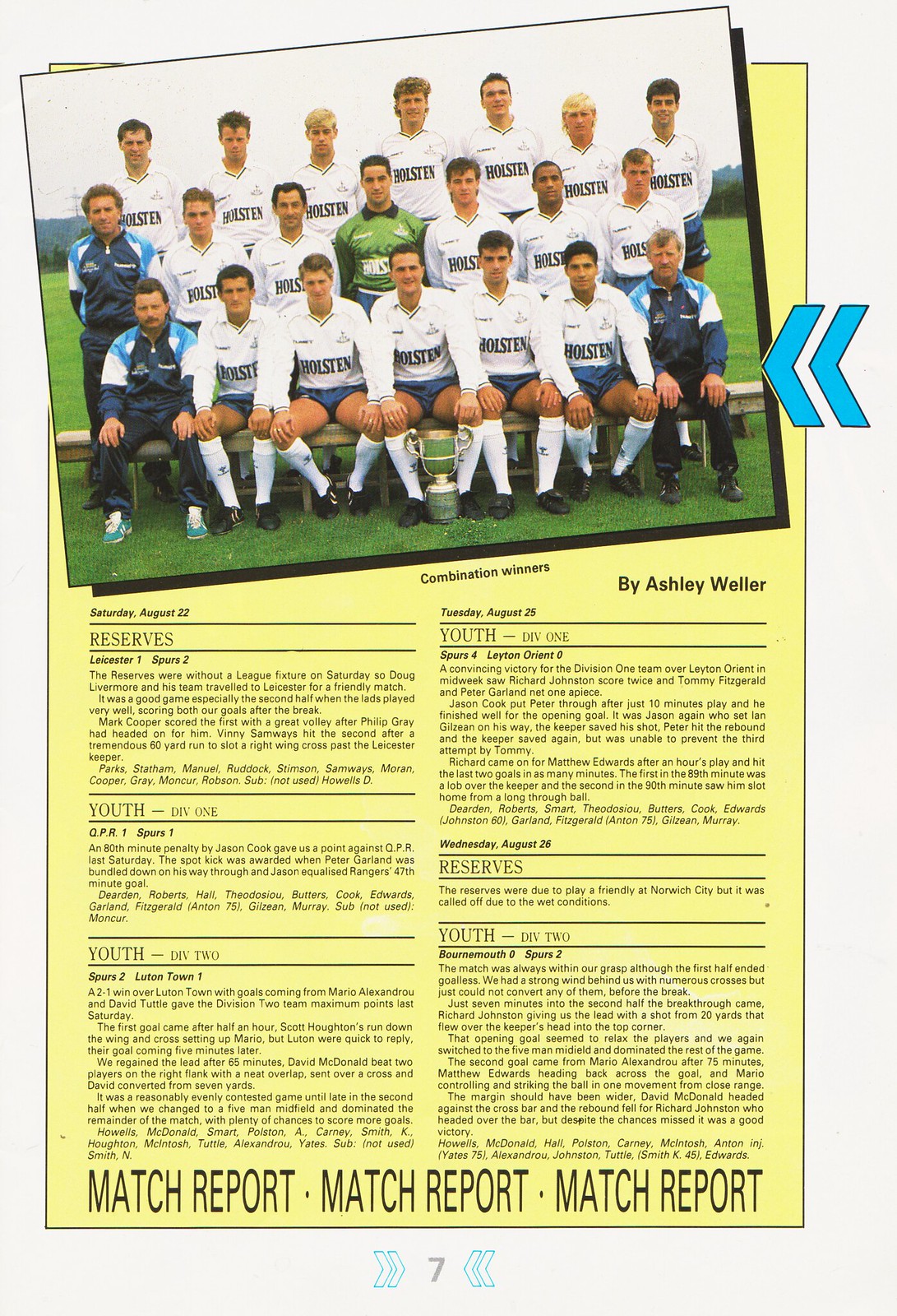This image is a visually dynamic page from what appears to be a program or magazine. It features a diagonally set, detailed photograph of a soccer team named Holstein. The team members are dressed in a standard uniform consisting of black shoes, white knee-high socks, blue shorts, and white shirts with collars—all emblazoned with "Holstein." Most players have short hair and are predominantly young to middle-aged. In the middle of the group stands a gentleman in similar attire, except his shirt is green, possibly indicating his significance, like a team captain or a key player.

Flanking him are three men—two on the left and one on the right—dressed in blue shoes, blue pants, and light blue and white jackets. These men likely serve as the coaches. Sitting conspicuously in front of the team is a large green cup trophy, reaching up to the center player's knee, indicating a notable achievement.

The text below the image is comprehensive, providing detailed event information. It lists key dates: Saturday, August 22nd for the reserves, youth division one, and youth division two; Tuesday, August 25th for youth division one, reserves, and youth division two; and Wednesday, August 26th also for the reserves and youth division two. The header "Combination Winners" followed by the caption “by Ashley Weller” highlights the article’s authorship. Additionally, it mentions a "match report" at the bottom and identifies that this content appears on page seven.